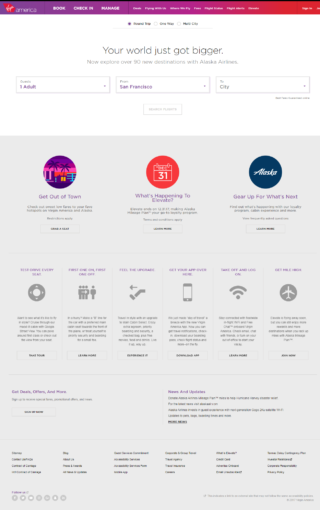The image depicts a screenshot with a visually striking, but somewhat chaotic and difficult-to-read appearance. A colorful banner spans the top, featuring vibrant hues of purple, pink, and orange, though the white text contained within it is unfortunately illegible. Below this banner lies a predominantly white background marred by extreme graininess and blurriness.

Prominently displayed text that can be deciphered reads: "Your world just got bigger. Now, explore over 90 new destinations with Alaska Airlines." Directly beneath this message are three distinct text boxes arranged horizontally. The leftmost box, adorned with purple text, indicates "One Adult." Adjacent to it, another segment in purple text specifies "San Francisco." The final segment prompts for a city but remains unfilled.

A light gray area below these boxes features three circular icons. The first circle contains a vibrant, digital illustration of a tropical scene with palm trees, buildings, and a sunset, accompanied by the text "Get out of town." The second circle showcases a calendar icon marked with the number 31, with the text "What's happening to elevate?" The rightmost circle, encased in a teal box, presents the word "Alaska" in clean white text.

Overall, the image attempts to convey a promotional message about new travel opportunities with Alaska Airlines, albeit through a somewhat cluttered and visually challenging presentation.